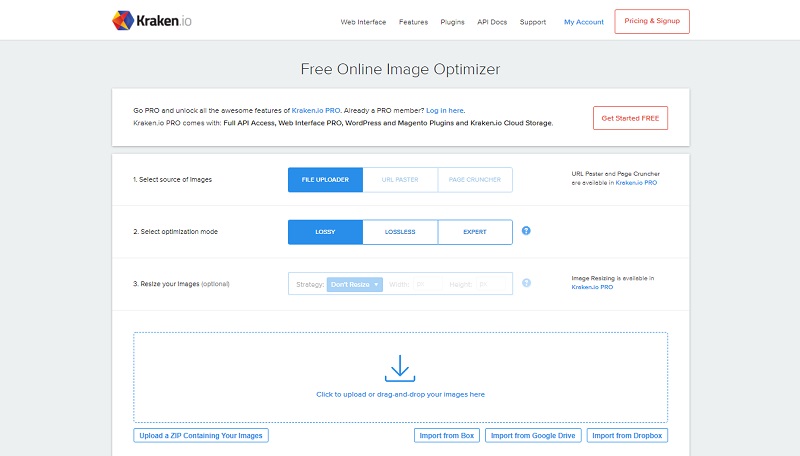Screenshot of the Kraken.io Website Interface:

At the very top of the screenshot, there is a logo featuring a blue hexagon with a yellow triangle on one side and a red triangle on an adjacent side. Next to the logo, the brand name "Kraken.io" is displayed, where "Kraken" is in black font and ".io" is in light gray.

Below the logo, there's a navigation bar with the following options: Web Interface, Features, Plugins, API Docs, and Support. To the right of these options, "My Account" is highlighted in blue font. Adjacent to this, a red outlined rectangle contains the words "Pricing and Signup" in red font.

The website's background is light gray. Prominently displayed is the title "Free Online Image Optimizer" in black font. Beneath this, a promotional message reads, "Go Pro and unlock all the awesome features of Kraken.io Pro. Already a Pro member? Log in here."

Further down, there is a button labeled "Get Started for Free." Underneath this button, options include File Uploader, URL, Lobby, and Expert. A sidebar to the right provides additional functionality with a downward arrow bracket icon and options including "Upload a Zip File," "Import from Box," "Import from Google Drive," and "Import from Dropbox."